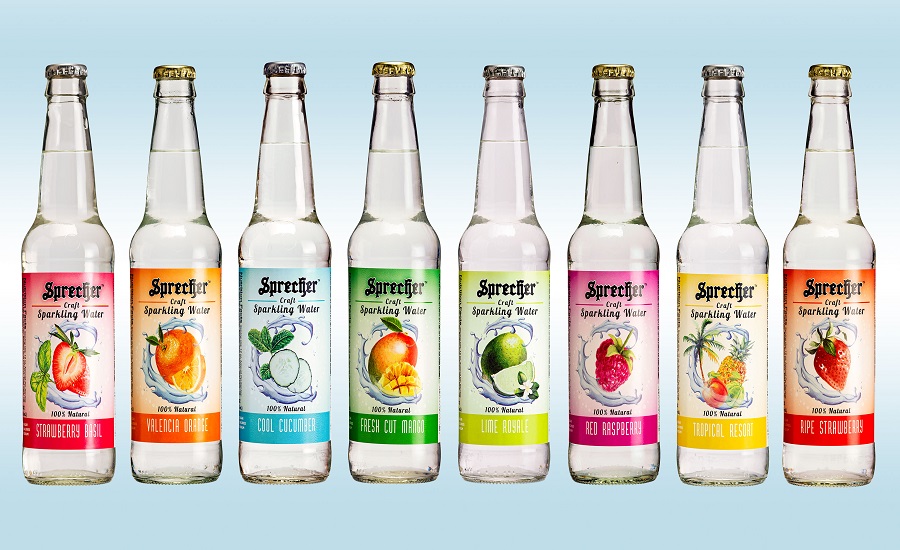This image showcases eight bottles of Britzifer craft sparkling water, each elegantly designed with a slender, long-necked glass body. The backdrop is a gradient of white in the center transitioning to light blue at the edges, providing a serene contrast to the vibrant labels adorning each bottle. The bottles are capped alternately with silver and gold tops, emphasizing their premium feel. All bottles are filled with clear, non-carbonated water, with labels specifically colored to match their respective flavors.

The flavors displayed are rich and varied: starting with two strawberry-flavored bottles, one with a pinkish label and the other a darker red, indicating a slight variation in the strawberry essence. Next in line is a Valencia orange flavor, followed by a striking blue-labeled bottle for blueberry. There's a fresh-cut mango flavor with a green label, a kiwi flavor with a lighter green label, a red raspberry flavor marked by a pinkish-purple label, and a tropical flavor featuring a pineapple on a bright yellow label.

Each label is brightly colored and features the fruit prominently, with "Britzifer" written at the top and "Craft Sparkling Water" below. This detailed array displays not only the diverse fruit flavors but also the meticulous design aimed at appealing to a sophisticated palate.